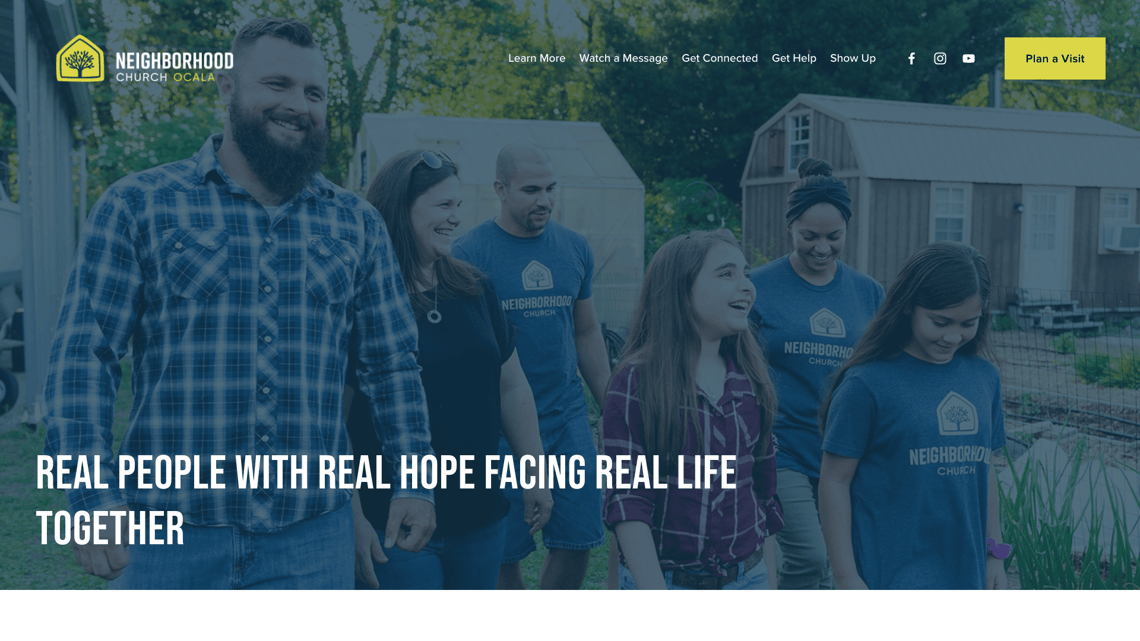In the image, a website titled "Neighborhood Church" is displayed prominently at the top left. To the right of the website title, there are five categories: "Learn More," "Watch a Message," "Get Connected," "Get Help," and "Show Up." Adjacent to these categories are icons for Facebook, Instagram, and YouTube. On the far right, a yellow button labeled "Plan a Visit" is visible.

Below this section, the image features six individuals viewed mostly from the front. On the far left stands a man wearing a white and blue checkered shirt, with his arms at his sides, sporting a beard and short hair, and smiling. Next to him is a woman in a black shirt and necklace with shoulder-length hair. To her right is a man dressed in a blue shirt. Positioned next is a child in a purple checkered shirt. Behind this child, a woman wearing a blue shirt can be seen. Lastly, another child in a blue shirt is present. The individuals in blue shirts have “Neighborhood” printed on their attire, likely indicating the church's branding. This group is situated in an outdoor environment, standing in front of what appears to be a shed and a barn, with a backdrop of abundant trees.

At the bottom left of the image, a caption in white text reads: "Real People with Real Hope Facing Real Life Together."